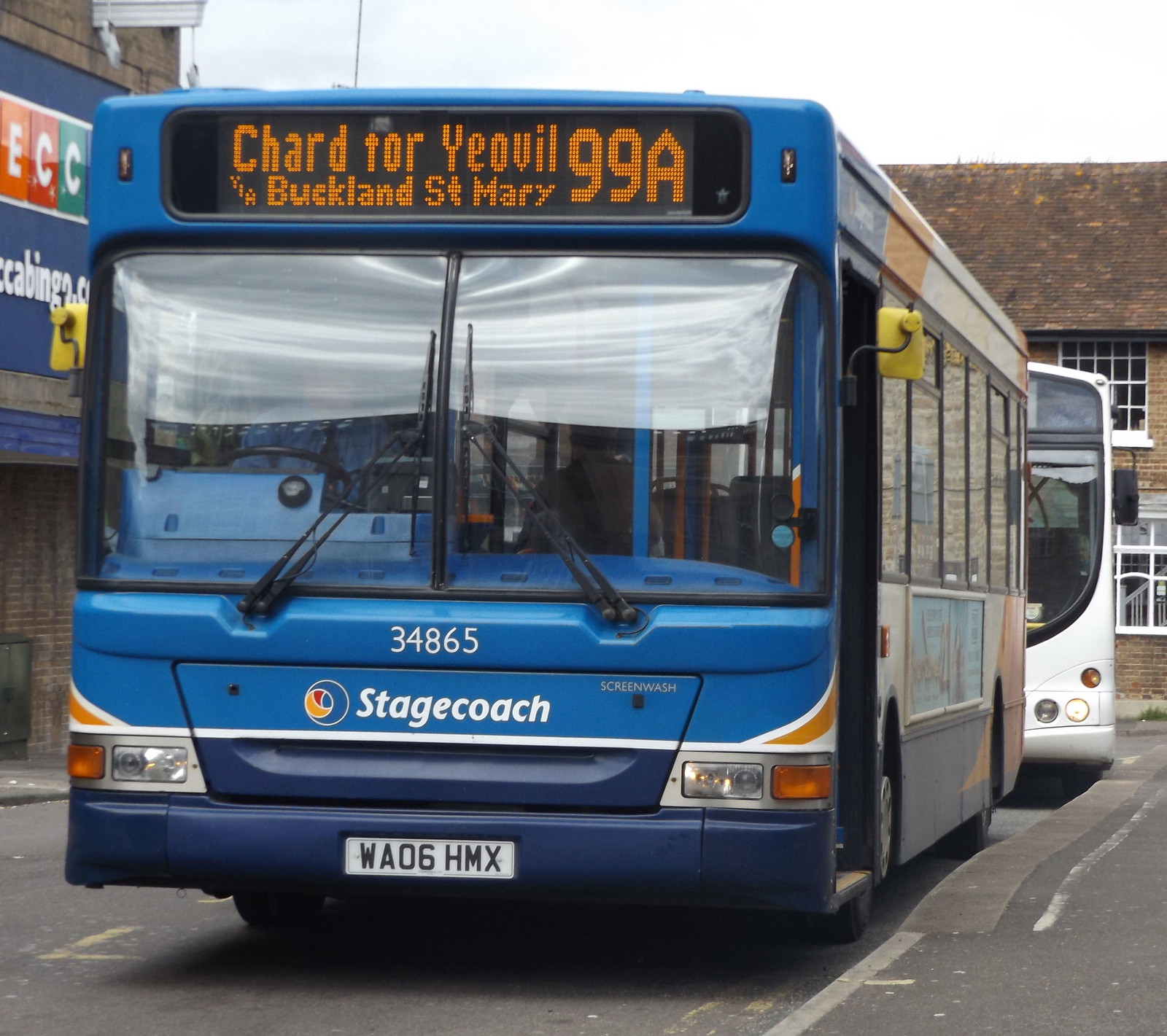This photograph captures a detailed view of a city bus on a road, likely in England, under a white sky with the background featuring some buildings with older shingled roofs and a partially visible billboard. Dominating the scene, a blue bus with orange trim is prominent. At the top front of the bus, a display screen in yellow letters reads, "Charred 4, Yeovil, Buckland St. Mary, 99A." The bus is branded with "Stagecoach" on the front bumper and the bus number "34865" is printed above this branding. The bus displays a license plate with the registration WA06HMX. The large windshield features two prominent window panes with substantial windshield wipers. Through the windshield, the driver is visible, seated at the right front of the bus. Behind this blue bus, there is a smaller portion of another white bus visible. The scene also suggests a cool, foggy daytime setting with no people in sight, reinforcing that these buses are parked in a lot.